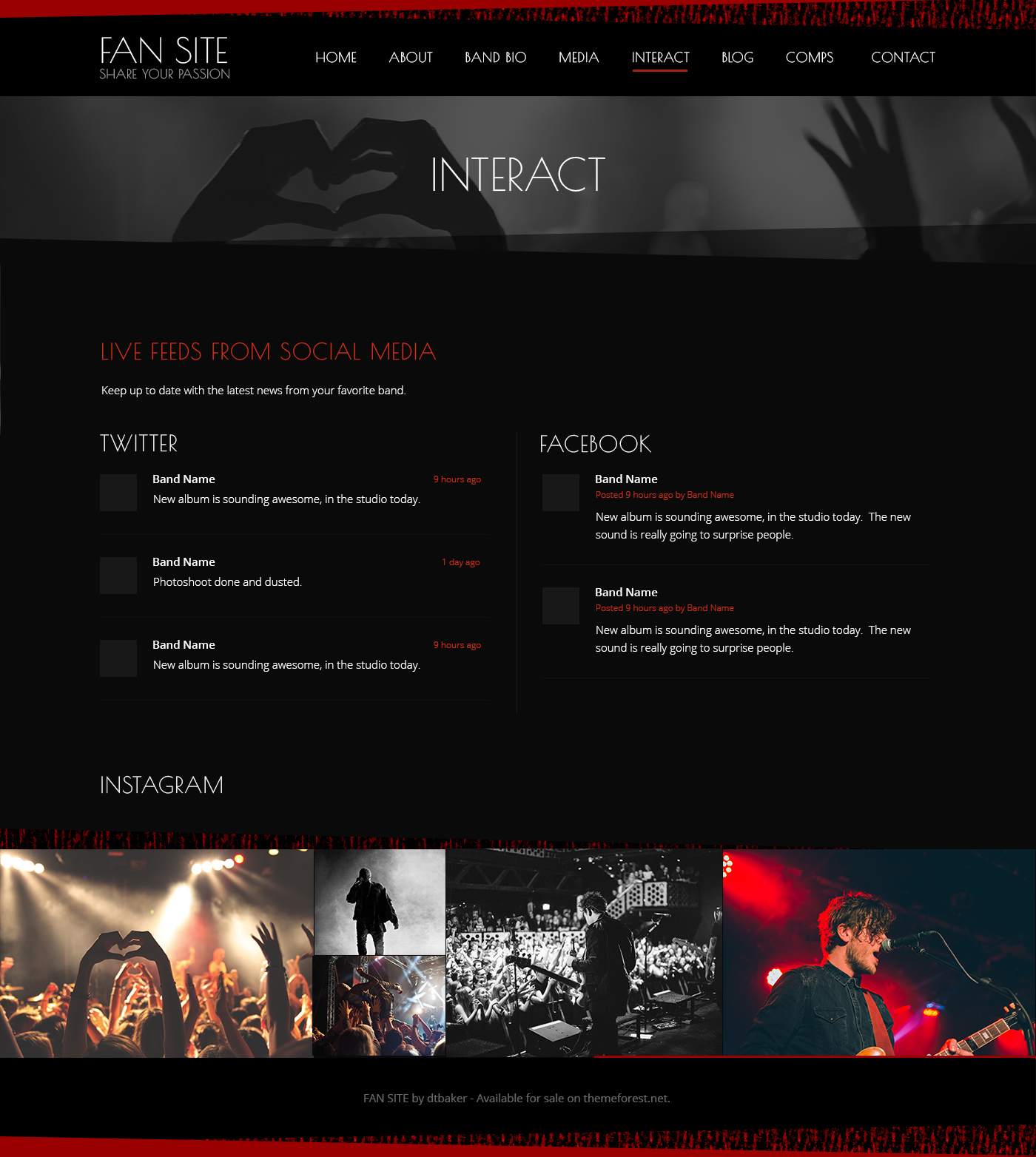In this website screenshot, the top portion features a bold red color, contrasting with a black background that occupies the lower half. The text is predominantly white, creating a striking visual effect. In the top left corner, the site is branded with "Fan Site: Share Your Passion." Adjacent to this, on the right, a series of navigational tabs are present: Home, About, Band, Bio, Media, Interact, Blog, and Contact. The "Interact" tab is underlined, indicating it is currently selected.

The section below the tabs features a background image of black silhouetted hands, creating a dynamic and engaging visual. To the left, the words "Live Feeds from Social Media" in red catch the eye immediately. Beneath this heading, a series of social media updates from the fan's favorite band is displayed in white text:

- "Keep up to date with the latest news from your favorite band."
- Twitter updates feature: "New album is sounding awesome in the studio today," posted nine hours ago, with the time in red.
- "Photoshoot done and tested," posted one day ago. 

Moving to the right, Facebook updates are shown:
- A post from nine hours ago reads, "New album is sounding awesome in the studio today. The new sound is really going to surprise people."

The Instagram section on the bottom left showcases vibrant images: fans making heart signs with their hands, performers on stage, and a guitarist at the microphone. 

At the very bottom of the page, a footer note states: "Fan Site by DT Baker available for sale on ThemeForest.net," with "ThemeForest.net" highlighted in red. The remaining text is in white, maintaining the visual consistency of the site.